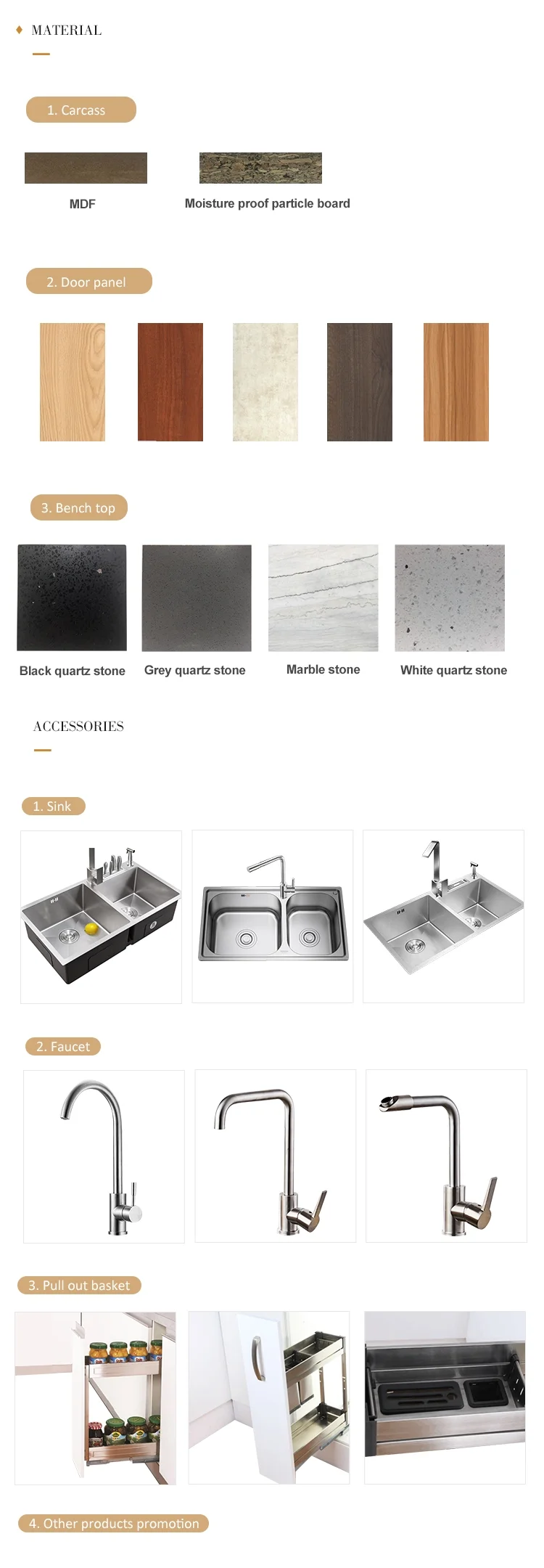On a stark white background, the word "MATERIAL" stands out in bold, black capital letters, accentuated by a small brown diamond and a brown line beneath the "M" and the "A." Below this header, a light brown banner bears the label "Number One Carcass," below which a series of colored rectangles and inscriptions are presented. 

First is a brown rectangle labeled "MDF," followed by a brown and beige marbleized rectangle marked as "Moisture Proof Particle Board." Below another light brown banner titled "Number Two Door Panel,” five different door panels are displayed: a blonde wood panel, a rosy dark brown wood panel, a beige whitewashed wood panel, a dark brown wood panel, and a medium brown wood panel.

Next, a light brown banner reading "Number Three Bench Top" features four examples: a black quartz stone, a gray quartz stone, a marble stone (with a distinctive gray and white swirl), and a white quartz stone speckled with gray.

Following, the word "ACCESSORIES" is depicted in black capitals with a brown line underneath. Then, under a light brown banner labeled "Number One Sink," three double sinks made of stainless steel are showcased. A subsequent banner titled "Number Two Faucets" displays three modern-looking stainless steel faucets.

Lastly, a light brown banner named "Number Three Pullout Basket" portrays cabinets equipped with a two-shelf pullout drawer, showing one on the left, one in the middle, and a top view of a shelf on the right. Below this, another light brown banner reading "Number Four Other Products Promotion" appears on the left, but it's cut off, transitioning into the untouched white background.